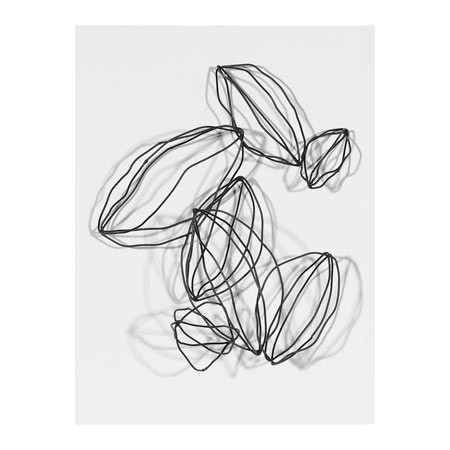The artwork is an abstract drawing on a plain white page, featuring seven overlapping shapes that resemble almonds, coffee beans, or lips, constructed out of either dark black or dark gray wire. These shapes vary in size and are arranged with three at the bottom right, two in the center, and two at the top right. The overlapping nature of the shapes makes the lines difficult to discern. The wire creates shadows that mimic the shapes, giving the illusion of a reflection or doubling the shapes, enhancing the complexity of the piece. The precise, intricate black and gray lines against the white background add to the abstract and ambiguous nature of the artwork, making it rich in texture and form.